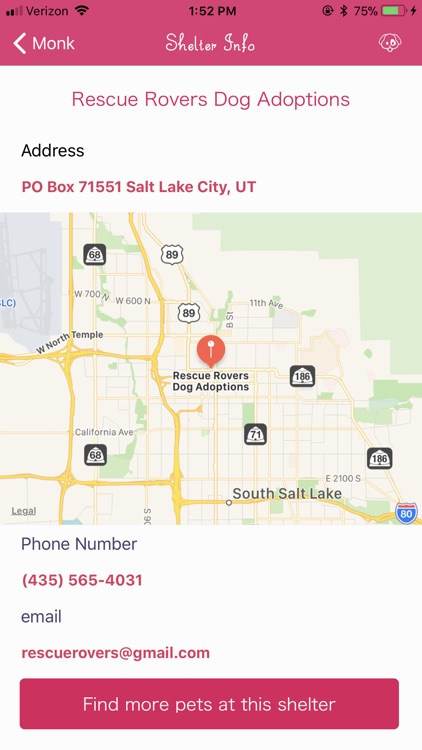The image features a smartphone screen interface with the following elements: 

At the top, a purple status bar displays "2 out of 4 bars," indicating signal strength, followed by "Verizon," the time "1:52 PM," a Bluetooth icon, and a battery indicator showing "79%."

Below the status bar, the title "Monk Shelter Info" is prominently displayed on a white background. Written in purple text beneath it, there's a heading: "Rescue Rover Dog Adoption," along with the address "P.O. Box 71551, Salt Lake City, Utah."

A Google Maps snippet is shown next, highlighting a red location pin labeled "Rescue Rover Dog Adoption." The map features parts of South Salt Lake and Interstate 80, though some details are not clearly visible.

Under the map, the contact information for the shelter is provided: phone number "435-565-4031" and email "rescuerover@gmail.com." At the bottom, there's a prominent purple rectangular button that reads "Find more pets at this shelter."